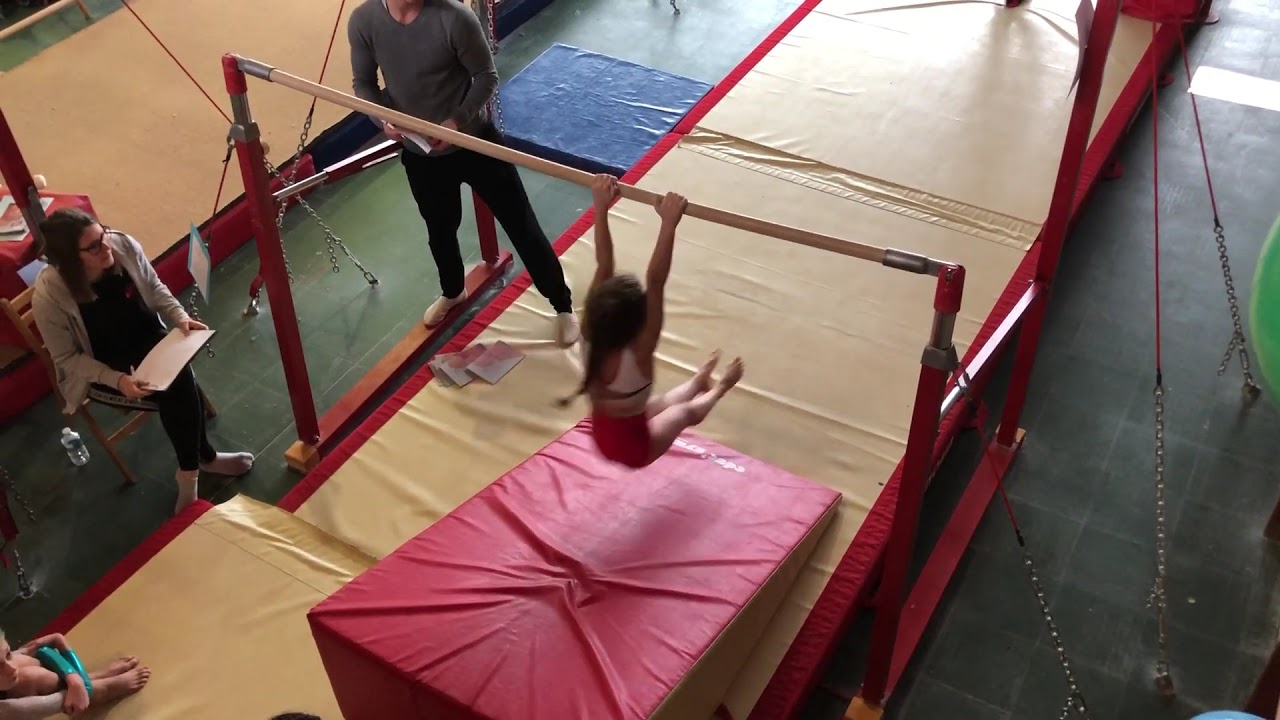The photograph captures a young gymnast, approximately three to seven years old, practicing in an expansive gymnastics studio. The image, likely taken from an elevated vantage point, shows the girl at the center, hanging from a light brown horizontal bar. Her small feet are outstretched in front of her, and her hair, a cascade of brown braids, trails behind her. She dons a red and white leotard, giving a vivid contrast to her back, which faces the camera. Directly beneath her is a large red foam mat, essential for safety, with surrounding lighter cream-colored padding bordered in red, forming what appears to be a runway.

To the left, two adults observe her movements intently. The woman, seated and donning glasses, wears a gray jacket over a black shirt with matching black pants and gray socks. She appears to be taking notes on the girl's technique, her gaze fixated while her hands clutch a sheet of paper or a notepad. Standing nearby is a man, his upper body cropped out of the frame. Clad in a tight-fitting gray shirt, black sweatpants, and white shoes, he too holds what seems to be a note card, possibly her coach assessing her form.

Additionally, a young girl, likely another gymnast, sits cross-legged at the bottom left of the image on the runway padding. Her legs, toes, and part of her arms are visible, indicating she is attentively watching the practice session. The scene is a quintessential snapshot of a young gymnast amidst training, under the watchful eyes of her coaches, encapsulated in an environment primed for skill development and safety.